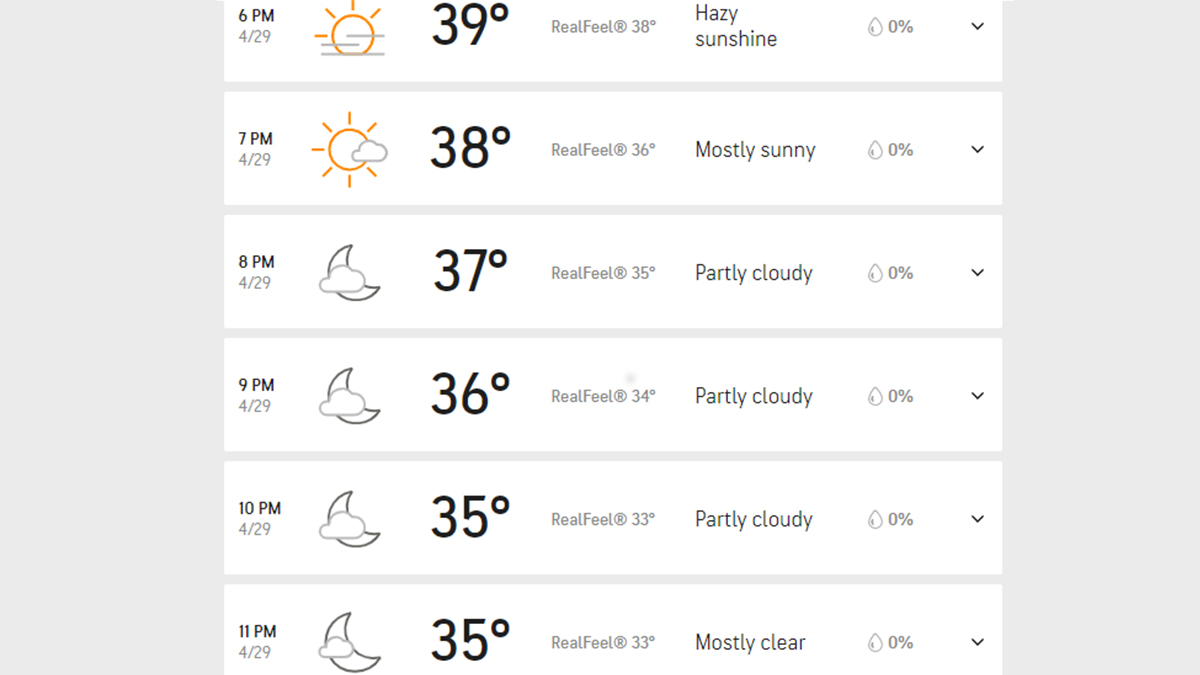This web page displays an hourly weather forecast for a specific but unspecified day. The projections span from 6 p.m. to 11 p.m. and are categorized as follows:

- **6 p.m.**: The symbol shows a sun, indicating hazy sunshine with a temperature of 39°F.
- **7 p.m.**: Mostly sunny conditions are forecasted with a temperature of 38°F.
- **8 p.m.**: The symbol depicts a partly cloudy sky with a cloud over a partial moon, with the temperature at 37°F. This pattern continues through:
  - **9 p.m.**: Partly cloudy with a cloud over a partial moon at 37°F.
  - **10 p.m.**: Partly cloudy with a cloud over a partial moon at 37°F.
- **11 p.m.**: Mostly clear skies are indicated with a cloud over a partial moon, and the temperature drops to 35°F.

Each time slot shows a detailed symbol and temperature forecast, gradually transitioning from hazy sunshine to mostly clear conditions as the evening progresses.